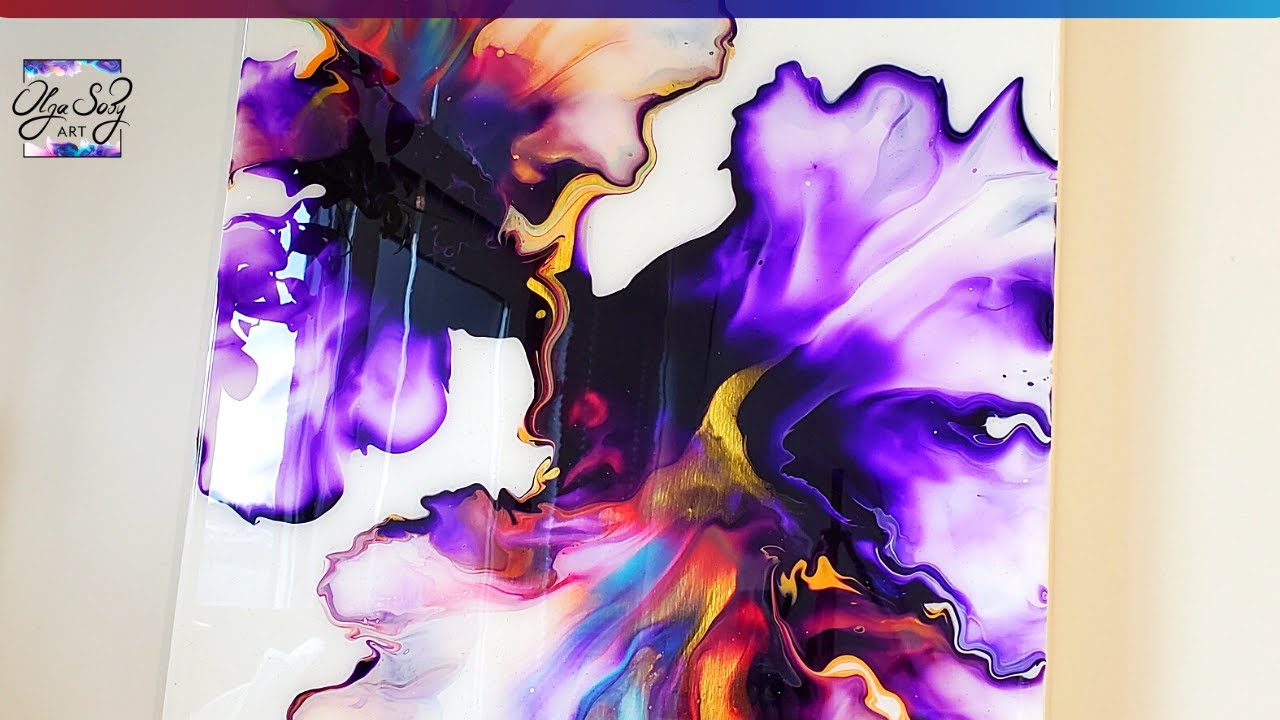This is an image of an abstract art piece with vibrant, fluid-like colors resembling watercolors flowing from a central point, resembling petals extending outward. The art features a striking palette of purples—ranging from deep to light—transitioning into gold, reds, and blues on a white canvas. The piece is propped against a cream-colored wall. At the top, a thin border transitions from deep red on the left to purple, dark blue, and finally, light blue on the right. In the upper left corner, the cursive watermark "OLGASOBYART" is visible. The overall composition has an organic quality with intricate gradations of color, imbuing the piece with a dynamic and vibrant character.